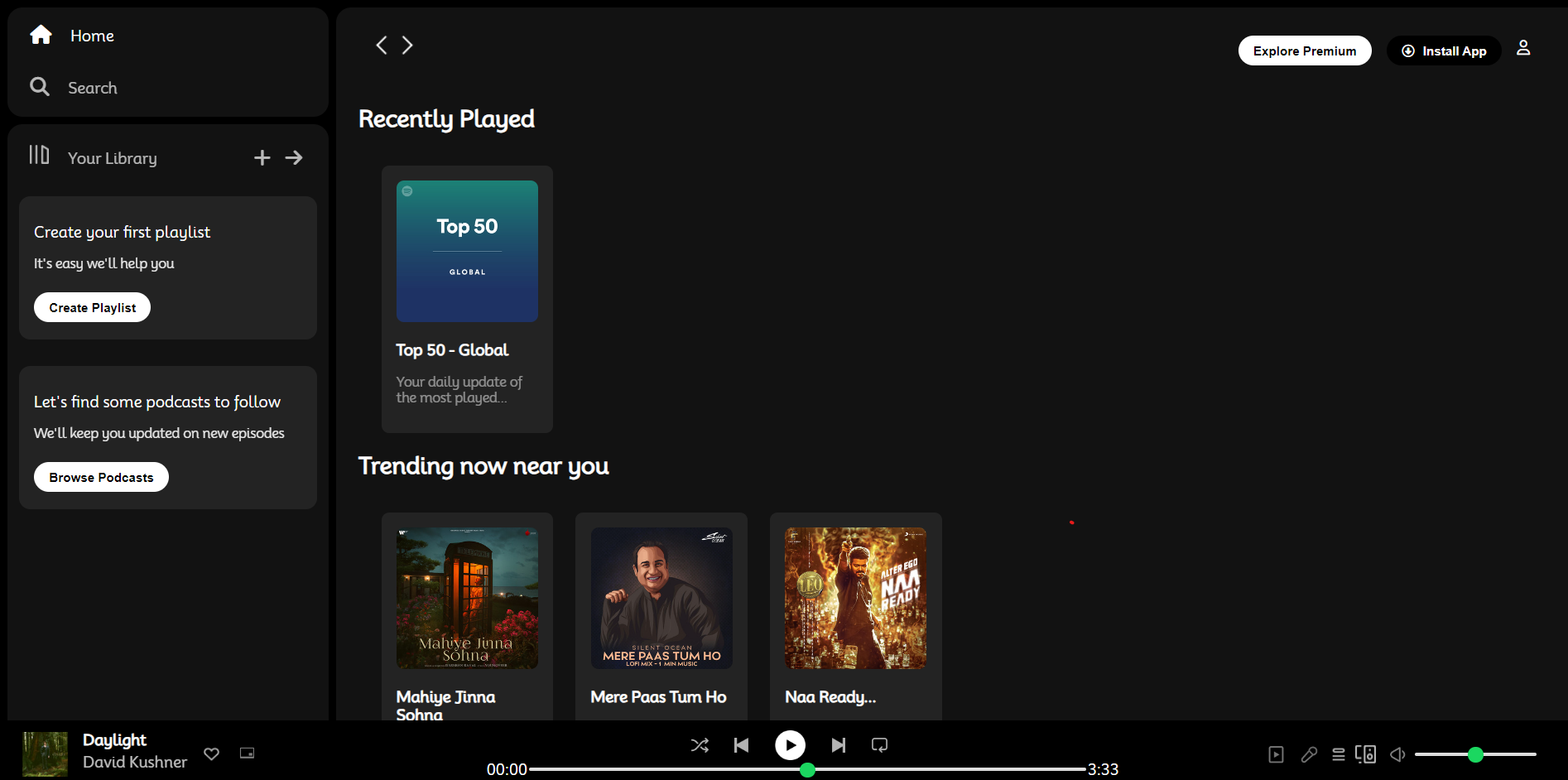This screenshot exhibits a black background, conveying a sleek and modern aesthetic. In the top right-hand corner, there is a white rectangle with rounded corners featuring the text "Explore Premium" in black. Adjacent to this, in white font against the black background, are the words "Install App." At the extreme corner, a small icon denotes an account profile.

On the left side of the image, a sidebar is visible. At the top of the sidebar, the word "Home" is accompanied by a white home icon. Directly below, the word "Search" is situated next to a circular search icon. Interestingly, the name of the website or streaming service remains unidentified.

Further down the sidebar, "Your Library" is indicated, offering two options. The first option, labeled "Create Your First Playlist," includes a clickable white button for initiating playlist creation. Below that, the prompt "Let's Find Some Podcasts to Follow" encourages users with the text "We'll Keep You Updated on New Episodes" and a clickable white button labeled "Browse Podcasts."

Towards the center-left of the image, three small images, likely album or song cover art, are displayed at the bottom. Above these images, a box with a blue background hosts the white text "Top 50." Beneath this, against the black background, the term "Top 50 Global" is prominently shown. This layout and content suggest the interface of a music streaming service, albeit unnamed.